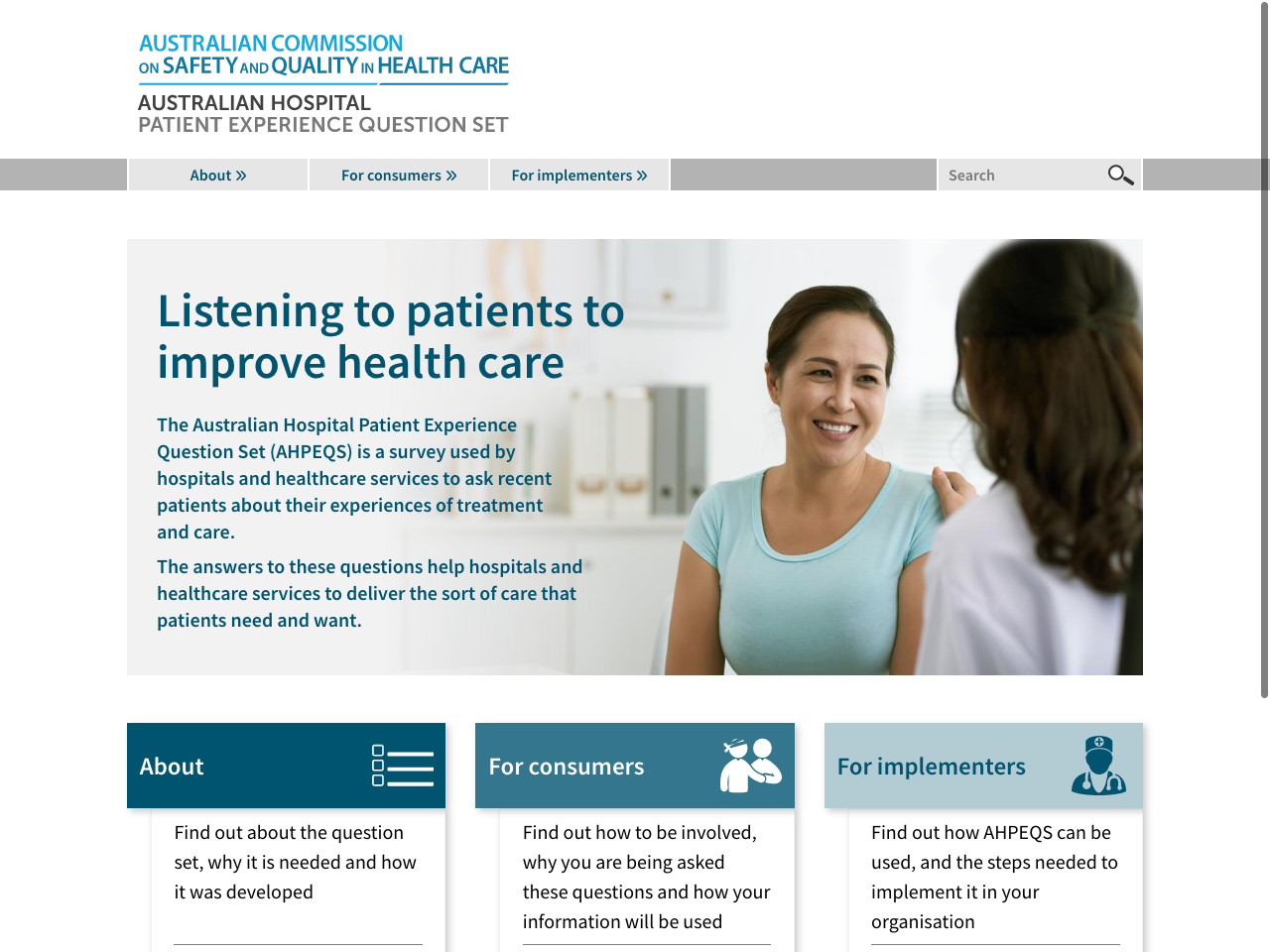**Caption:**

The top of the image features the text "Australian Commission on Safety and Quality in Health Care" with a line underneath. Below, it reads "Australian Hospital Patient Experience Question Set" next to a search bar. The main image depicts a doctor conversing with a woman, emphasizing the importance of listening to patients to improve healthcare. The Australian Hospital Patient Experience Question Set is a survey conducted by hospitals and healthcare services to gather feedback from recent patients about their treatment and care experiences. The responses to these questions enable hospitals and healthcare services to provide the type of care that patients need and desire. The image contains additional text inviting readers to learn more about the question set, its necessity, and its development. For customers, it provides information on how to get involved, why these questions are being asked, and how their information will be used. For implementers, it offers guidance on how the question set can be utilized and the steps required to incorporate it into their organization.